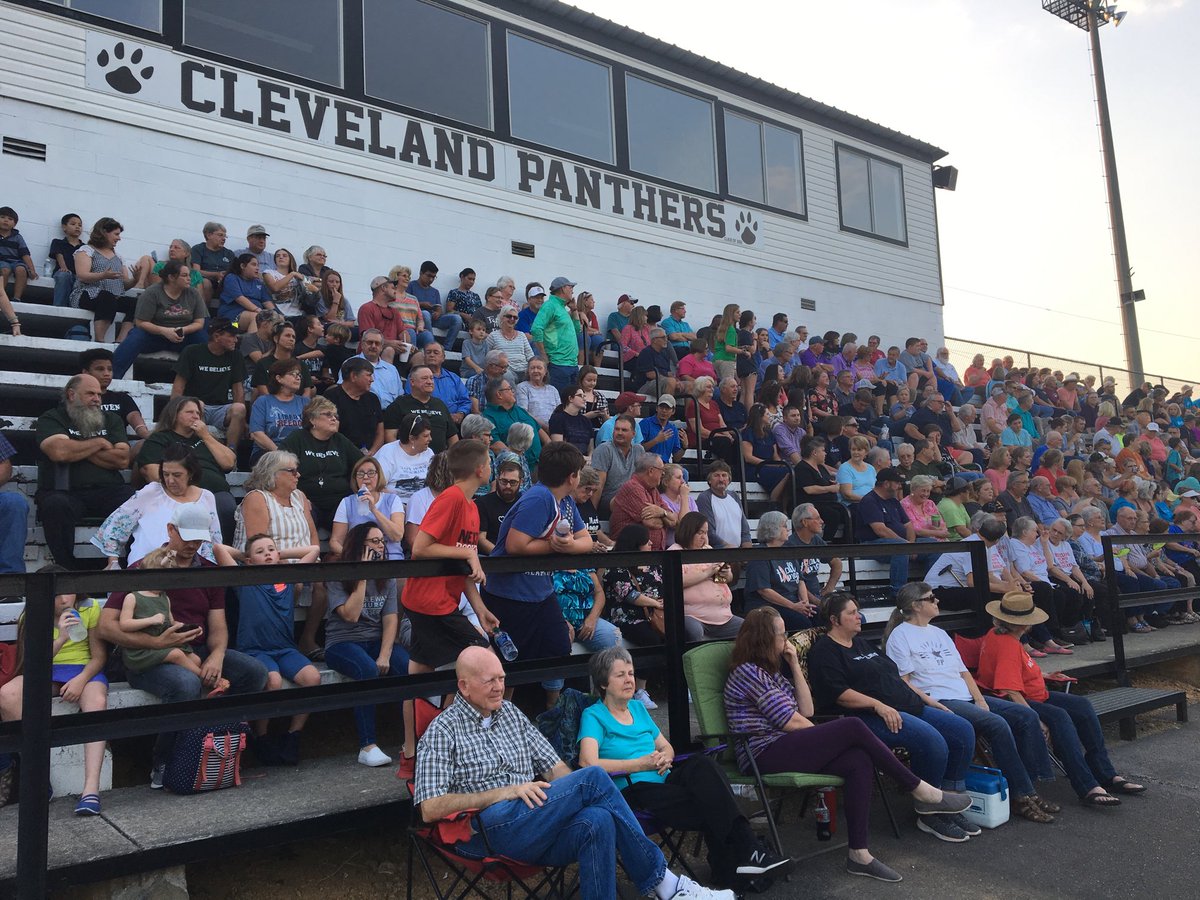In this vibrant image, a diverse crowd fills the bleachers at a Cleveland Panthers sporting event. Positioned behind and above the bleachers is a white press box with numerous windows overseeing the action. Below these windows, a sign boldly displays "Cleveland Panthers," flanked on each side by paw print silhouettes. A tall spotlight tower looms to the right, extending up to the top of the image. The bleachers, which appear to be whitish in color, are framed with black railings at the front. In the foreground, additional spectators are seated in set-up chairs. The crowd itself is a colorful tapestry, featuring people of all ages—from children to grandparents—adorned in a variety of hues, including blues, reds, greens, pinks, whites, and blacks. There's a notable group in the front row wearing matching shirts, suggesting they belong to the same organization. Despite the excitement of the scene, many in the crowd appear to be engaged in conversation, indicating a lull in the on-field action. The sky overhead is a bright, almost white, backdrop to this snapshot of community and sportsmanship.